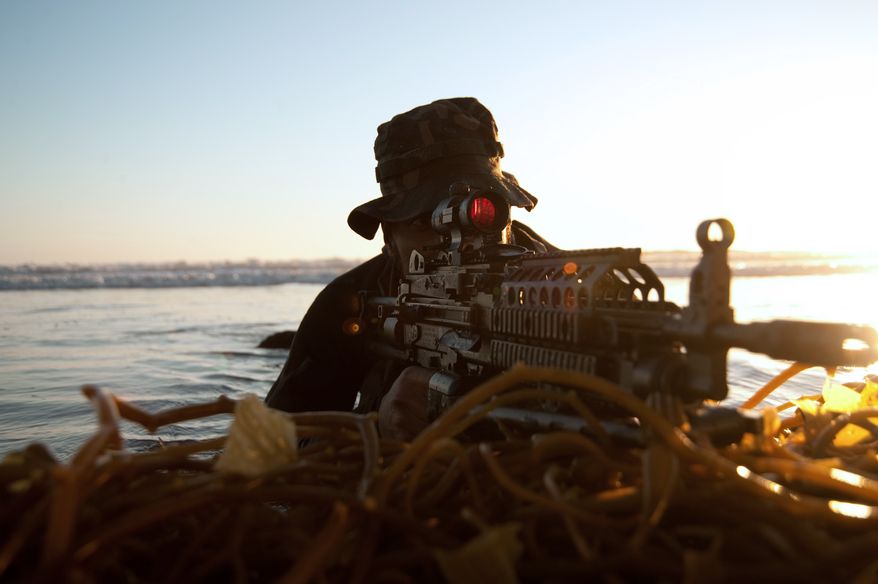In this high-resolution landscape photograph, a figure, whose identity is obscured by a camouflaged bucket hat, is poised with a substantial and sophisticated firearm equipped with optical lenses and a red scope. The gun, a precise and deadly large machine gun, is aimed just to the right of the viewer, implying a potential target off-frame. The person, potentially a soldier, is either laying or sitting in water, surrounded by seaweed or algae, effectively using the environment as natural camouflage. This backdrop includes a large body of water, possibly a lake, ocean, or river, with the distant sun illuminating a clear blue sky. The scene captures a moment of intense focus as the individual looks through the sight of the weapon, finger on the trigger, blending seamlessly into the aquatic and vegetative surroundings, which may serve as a makeshift barricade.